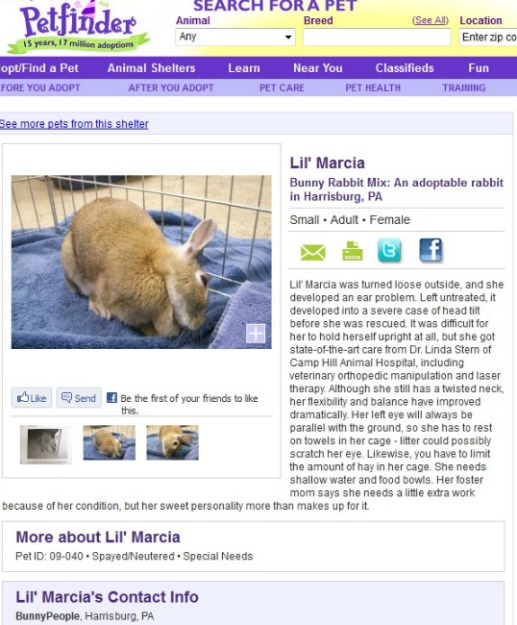This screenshot captures the homepage of a website dedicated to pet adoption.

In the upper left corner, the site features its title and logo in purple text: "Pet Finder." Directly beneath the logo, a wavy green banner displays the message "15 Years, 17 Million Adoptions" in purple text.

To the right of this banner, there are three interactive search boxes. The first box is a dropdown menu labeled "Animal," allowing users to select a specific type of pet. The second box is for "Breed," enabling detailed searches based on pet breeds. The third and final box, labeled "Location," invites users to enter their zip code to find pets near them.

Above these search boxes, bold purple text reads "Search for a Pet," guiding users through the initial steps of the adoption process.

The navigation menu, set against a black and purple background, spans the width of the webpage. It includes menu items: "Find a Pet," "Animal Shelters," "Learn," "Near You," "Classifieds," and "Fun."

In the upper left area of the image, there is a color photograph of a tan bunny rabbit lying in a tan-colored cage. The rabbit is comfortably resting on a blue towel.

The overall design and layout of the website aim to facilitate the search and adoption of pets while emphasizing its long-standing commitment and success in animal welfare.